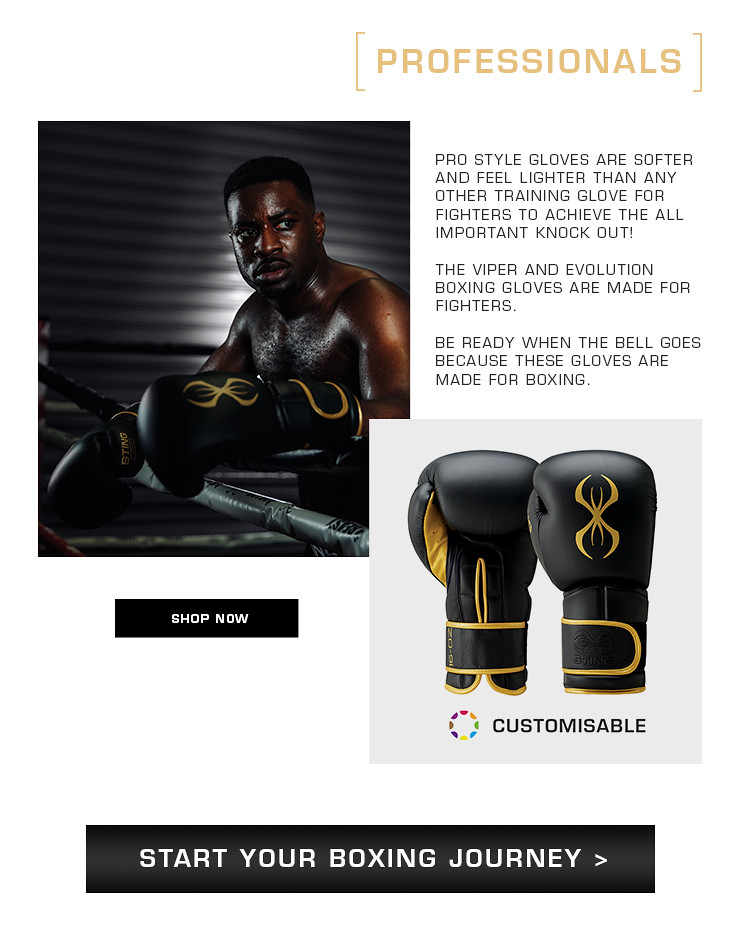This is a detailed advertisement image for professional boxing gloves. The ad has a white background with green uppercase text in the upper right corner that reads "PROFESSIONALS." Prominently featured is a black gentleman, very sweaty, as if he is in the middle of a fight or resting between rounds. He is wearing a pair of black boxing gloves with yellow accents along the edges and inside, adorned with a spider-shaped logo, indicating the Viper and Evolution models. 

The promotional text beside him states, “Pro-style gloves are softer and feel lighter than any other training glove for fighters to achieve the all-important knockout. The Viper and Evolution boxing gloves are made for fighters. Be ready when the bell goes, because these gloves are made for boxing.” The advertisement emphasizes customization, suggesting that their colors can be changed according to personal preference.

Below the descriptive text is a close-up image of the gloves: the glove on the left is shown from the front, while the glove on the right displays the backside with the distinctive spider-like design. Towards the bottom of the image, a black rectangular box contains the white text "SHOP NOW," urging immediate purchase. Further, there is another call-to-action in a larger gray rectangle with white text that reads, “START YOUR BOXING JOURNEY,” accompanied by a directional arrow pointing to the right.

In summary, the advertisement effectively combines images and text to highlight the features and appeal of these customizable, professional-grade boxing gloves.